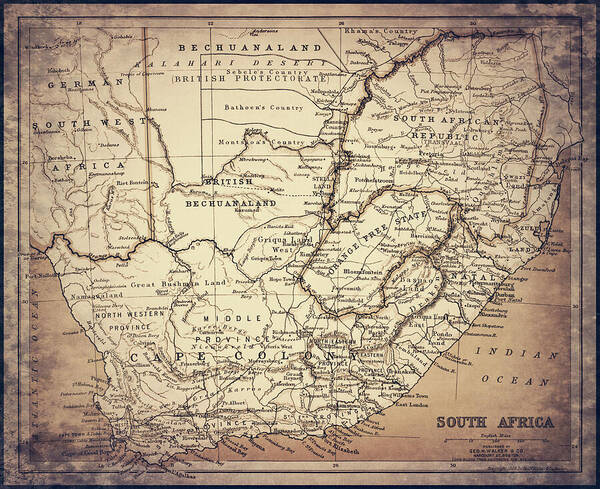The image is an old map of South Africa rendered in light brown and beige tones, suggesting an aged or antique appearance. It includes potentially decorative shading in the four corners, which might be mistaken for mold. Labelled prominently in the bottom right-hand corner is "South Africa," with "Indian Ocean" written above it. On the left-hand side, "Atlantic Ocean" is clearly legible, while the top center features the labels "Bishwan" or "Bechuanaland," "Alahari," and "Kalahari Desert," with "British Protectorate" in parentheses. The upper left corner is marked "German Southwest Africa." Various regions and landmarks are denoted across the map, including "Cape Cod," "Northwest Province," "Middle Province," "Orange Free State," "South African Republic," and another instance of "Bechuanaland." However, much of the map’s text is difficult to read due to the small lettering.